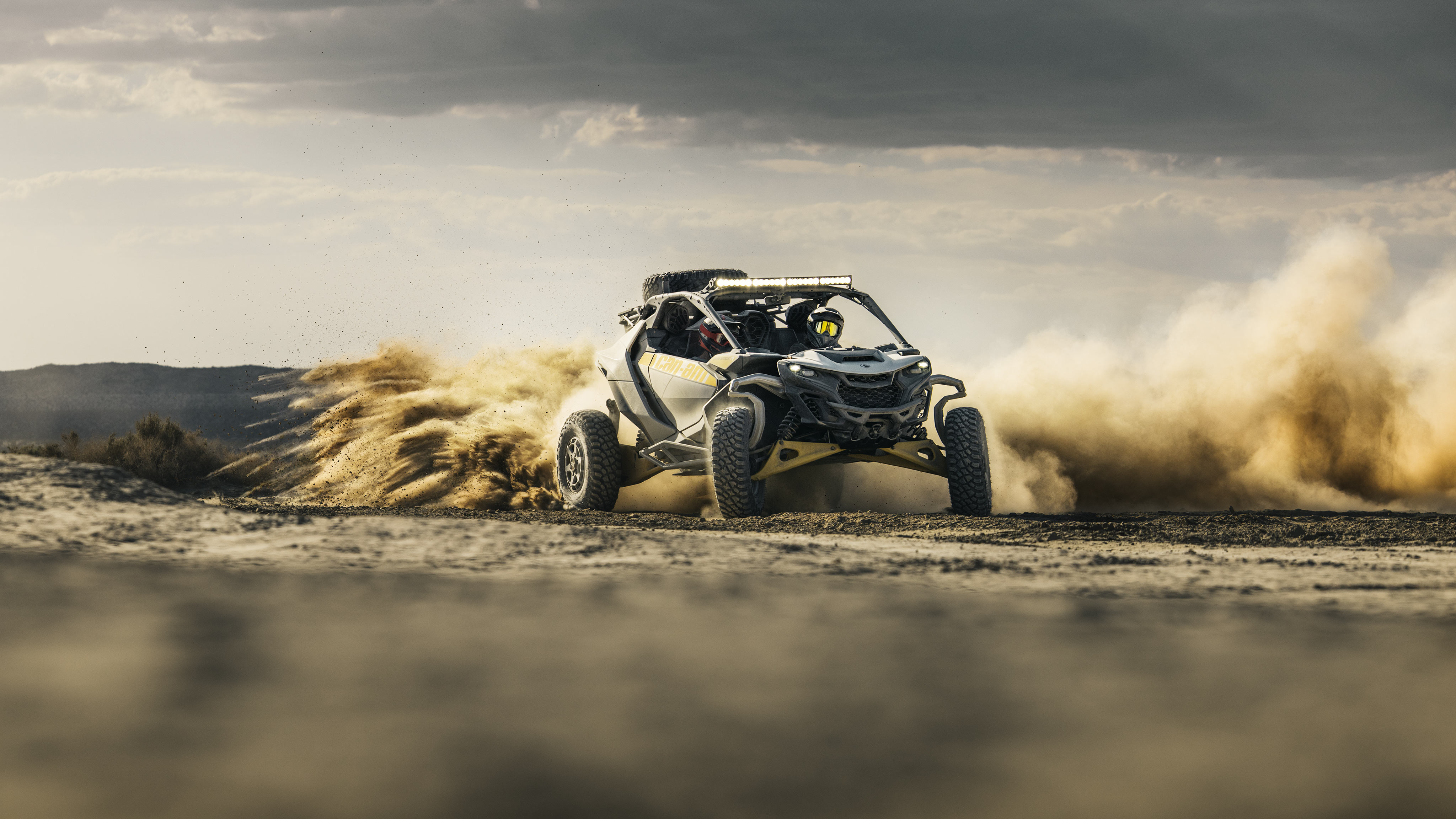In this image, an advanced off-road race car, resembling a high-tech dune buggy, is captured in the midst of an intense and exhilarating maneuver. The vehicle, primarily gray with yellow accents and large black wheels, appears to have just executed a high-speed, sharp turn, kicking up a substantial cloud of dust and sand that trails dramatically to the left. The driver, wearing a race helmet with reflective goggles, is visible in the seat, embodying the adventurous spirit of the scene. This exciting moment is set against a backdrop that features a partially clear blue sky with patches of dark clouds, low-lying hills, and sparse brush. The blurred foreground and additional hints of tumbleweed emphasize the motion and ruggedness of the desert-like terrain.